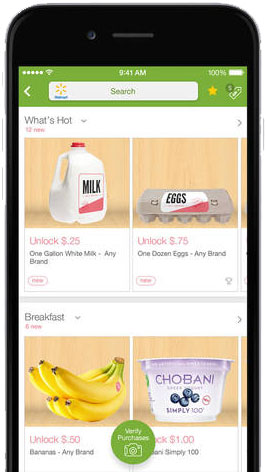This image captures a smartphone displaying the Walmart app interface, suggesting a user-friendly layout typical of advertisement photography. Dominating the screen is the app's distinct green menu bar at the top, indicating full Wi-Fi connectivity, network service, a fully charged battery (100%), and the current time at 9:41 AM. 

The central Walmart logo, consisting of a yellow sunburst followed by blue squiggly lines that spell "Walmart," is prominently visible. Below the search bar, various promotional icons are displayed, including a yellow star, a sale tag, and a "What's Hot" section featuring images of groceries: a gallon of milk, a carton of eggs, bananas, and a cup of blueberry Chobani yogurt.

Further details reveal this is a cashback app interface, possibly Ibotta, offering specific cashback rewards for purchasing certain items at Walmart. The offers listed include $0.25 back for one gallon of whole white milk (any brand), $0.75 back for one dozen eggs (any brand), $0.50 back for bananas (any brand), and $1.00 back for Chobani Simply 100 yogurt. The phrase "verify purchase" indicates the steps needed to claim these offers, emphasizing the app’s purpose of providing users with monetary rewards for shopping.